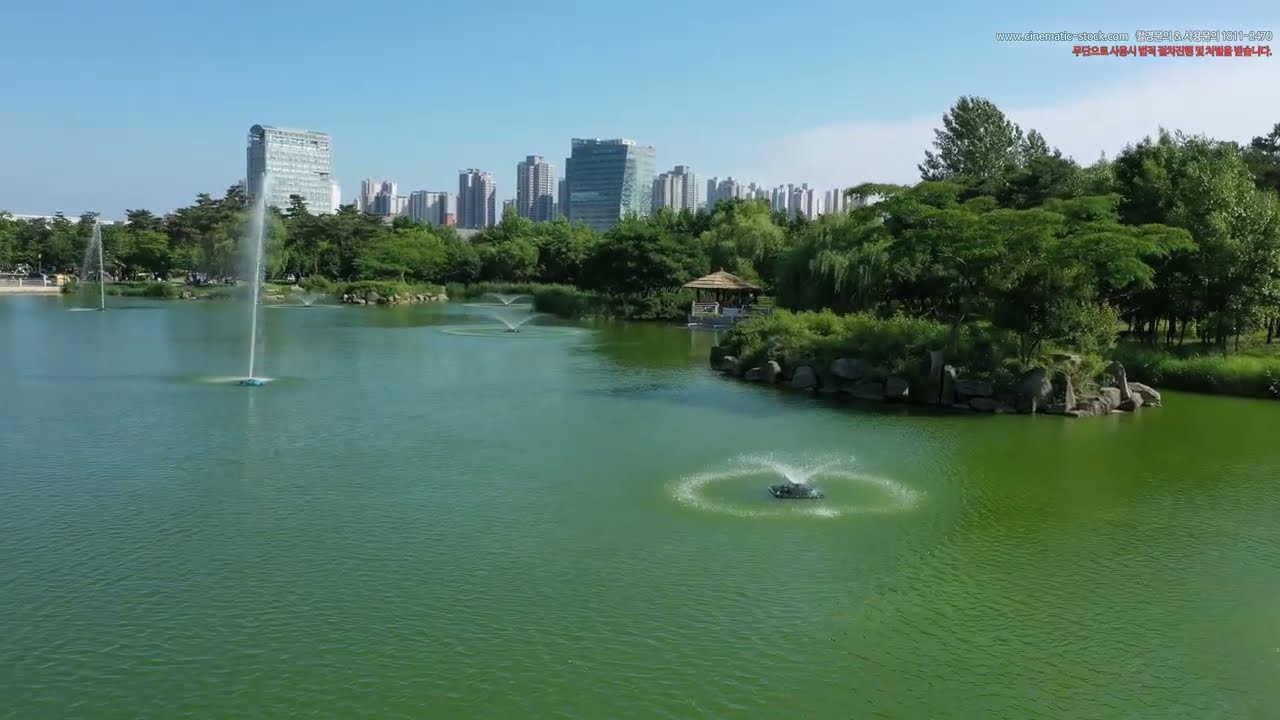The image is a daytime, color photograph taken from above, showcasing a scenic outdoor landscape. The prominent subject is a body of greenish water adorned with multiple fountains, each shooting streams of water in various patterns—some straight up into the air, others fanning out in a V-shape. This water body, possibly a river or lake, spans the lower half of the image. Surrounding the water is a lush, green shoreline with tall trees and grass. A pagoda overlooks the water from one side. 

In the background, the urban skyline features numerous skyscrapers in shades of gray and beige, with many windows reflecting the clear blue sky. The sky itself is predominantly blue with a few white clouds in the upper right corner. 

There's a watermark in the top right corner that reads "cinematicstock.com" in white text along with foreign characters—an overlay of Asian text in white and red, suggesting it might be used for digital wallpaper. The overall scene is absent of people and animals, focusing purely on the tranquil interaction between nature and urban elements.